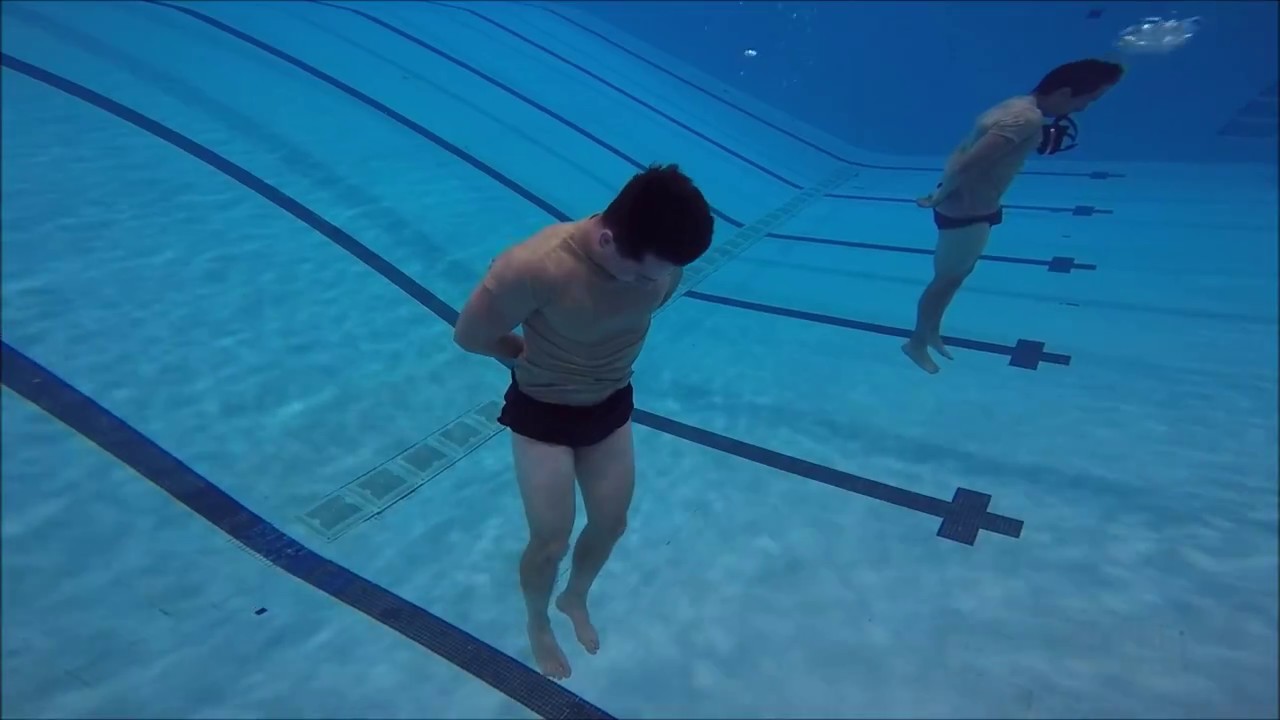In this image taken underwater in an indoor swimming pool, two divers, both wearing swim trunks, are captured descending into the deep end. The scene is bathed in varying shades of blue, characteristic of chlorinated pool water, with the divers’ flesh providing a stark contrast. Both men seem to be holding their breath as they have not yet reached the pool's bottom, evident from the bubbles trailing from one of them. The pool's design is reminiscent of an Olympic pool, featuring distinct lines at the bottom indicative of lane markers, and a noticeable slope transitioning from shallow to deep. In the foreground, one diver's legs and torso are visible, with some ambiguity surrounding potential folds of skin or a loose shirt. The background reveals another diver, who seems to be equipped with a camera in their mouth, suggesting they might be documenting the descent. The pool’s infrastructure includes white lines crossing its width, possibly related to filtration or demarcation. The photograph highlights the serene yet dynamic environment of underwater exploration in a controlled, indoor aquatic setting.